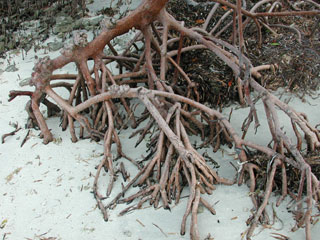The photograph depicts a snowy landscape dominated by an intricate network of tree roots and branches, both dead and intertwined. The scene is set on uneven terrain, perhaps indicative of a mountain slope, characterized by mottled white snow blanketing the ground. The composition is centered around a main root that twists from the middle top of the image to the bottom right, with numerous smaller roots and branches fanning out in various directions. These roots and branches, varying in size, create a complex web that both lays atop and partially sinks into the snow. The branches are predominantly pale brown with some darker hues near the center. Additional details include small sticks scattered around the main roots and slight greenery at the top left, providing a subtle contrast to the otherwise stark white background. At the top right, a sparse shrub of brown adds further texture to the scene. The overall effect is a striking juxtaposition of organic forms against a pristine, snowy backdrop.